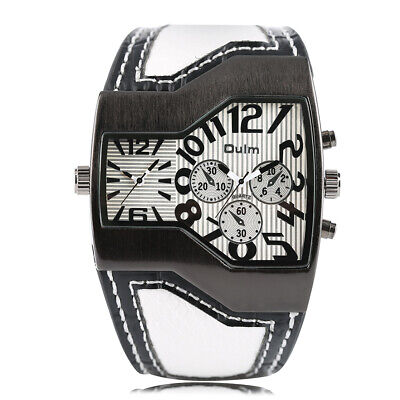The image showcases a striking black, white, and gray wristwatch designed like a thick, bracelet-style timepiece with a deep dark brown leather strap adorned with top stitches of white thread. The watch, central in the image, features multiple dials and gauges, creating a complex and sophisticated appearance. Main features include three smaller, possibly pressure gauges or secondary timekeeping dials, alongside a larger primary dial. Each dial has a distinct design; the smaller ones have horizontal stripes, while the larger one displays vertical stripes. The watch face is marked with bold, easily readable numbers. Additionally, there are several knobs suggesting that each dial can be adjusted independently. The background of the image is white, highlighting the watch, and the whole setup suggests a professional product photograph, likely intended for advertising. The brand name "O-U-L-M" is subtly present on the watch, though finer details remain too small to discern clearly.